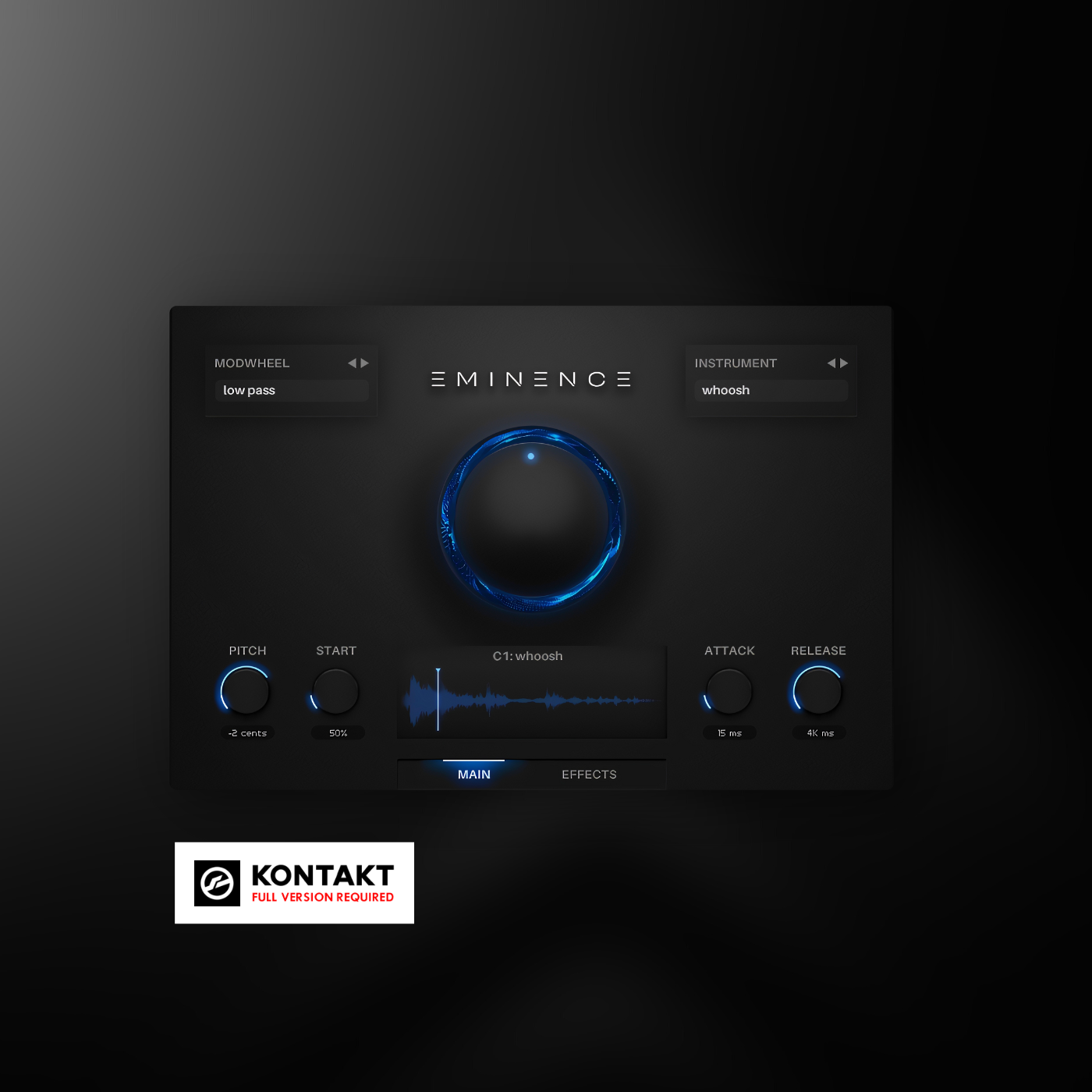This detailed CGI image depicts the user interface of a Kontakt software plug-in called Eminence, designed for use in digital audio workstations (DAWs). Prominently centered at the top, the name "Eminence" is displayed above a striking blue, light-filled knob surrounded by swirling light or water, with a tiny blue dot at the top, potentially indicating volume or spatial direction. The interface showcases various controls, including pitch, start, attack, and release dials at the bottom. A central waveform with a bright line traverses across it, hinting at the movement and decay of sound. To the left, under "Modwheel," you can see a lowpass filter with forward and backward arrows. On the right, under "Instrument," labeled "Woosh," are similar navigation arrows. A lit-up bar over "Main" juxtaposes against an unlit "Effects" tab nearby, and on the far right are additional knobs for attack and release. This sophisticated tool is integral for movie music composition and sound mixing, set against a charcoal background with a black interface, and requires the full version of Kontakt to operate.